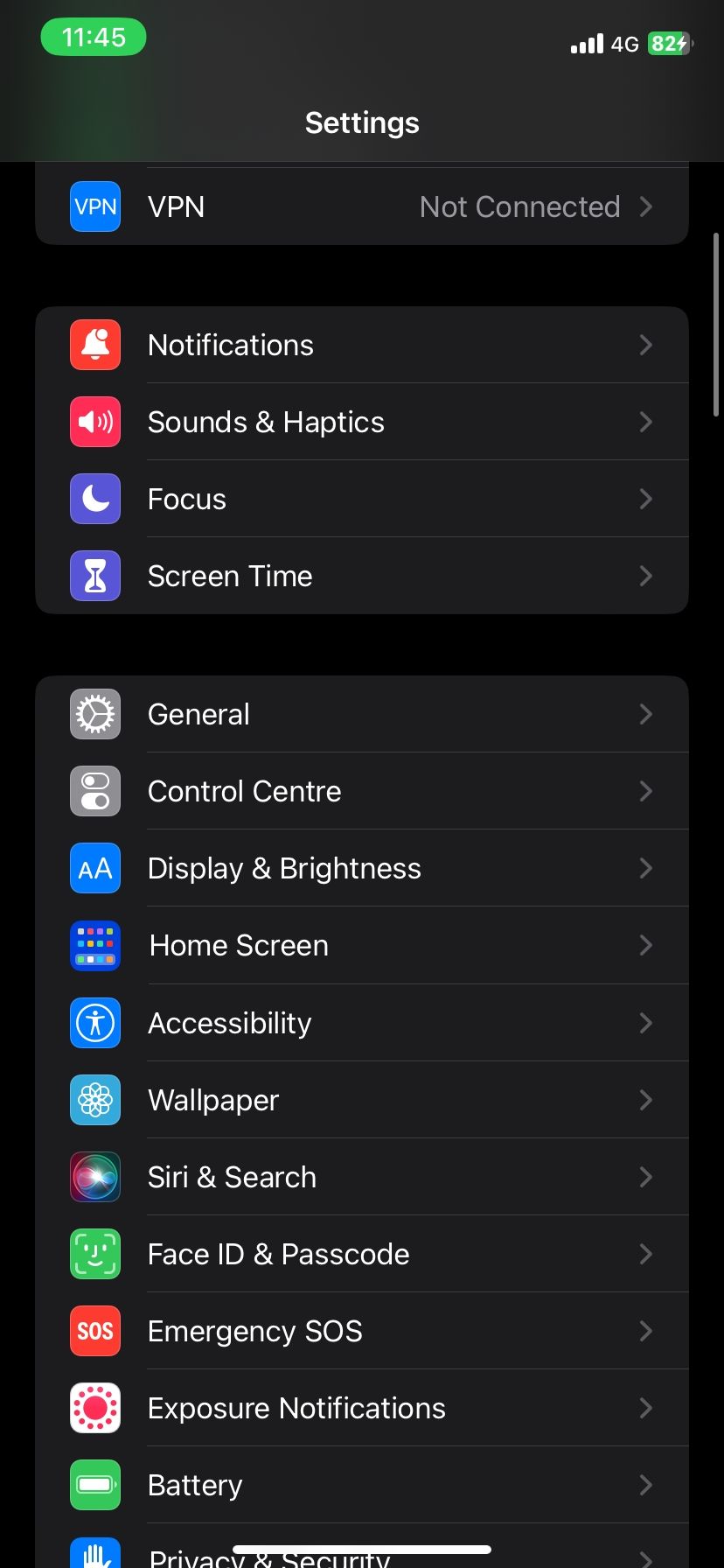This is a screenshot of the settings panel on an iPhone, displayed in Night Mode, which gives the screen a predominantly black background. At the top left corner, the time is shown within a green oval shape, indicating that the user was on a call while taking this screenshot. The top right corner displays the phone's signal strength and battery icon. Centrally located at the top, there's the word "Settings" to denote the current menu. Below this header, a vertical list of settings options is visible, each accompanied by a rightward-pointing arrow to expand respective categories.

The uppermost entry is labeled "VPN," with the status displayed as "Not Connected" to its right. Following this, the list includes: Notifications, Sounds & Haptics, Focus, Screen Time, General, Control Center, Display & Brightness, Home Screen, Accessibility, Wallpaper, Siri & Search, Face ID & Passcode, Emergency SOS, Exposure Notifications, and Battery. The bottom of the screenshot indicates that the list can be scrolled further to access additional settings.